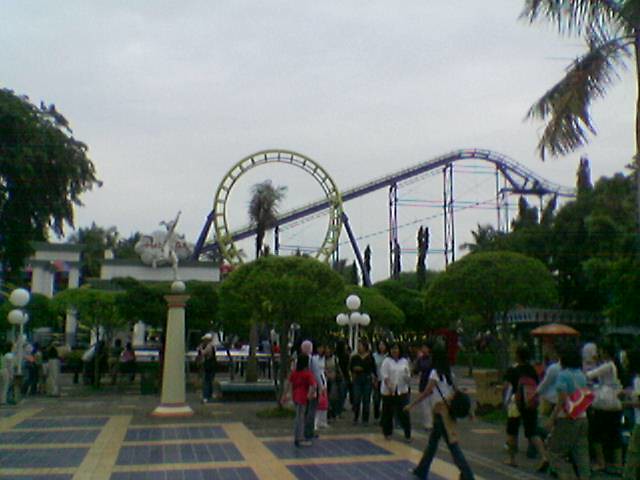This photograph captures the bustling entrance of an amusement park, characterized by a colorful tiled walkway with blue and yellow patterns. At the end of the walkway, a tall green pedestal supports a silver statue of a child kicking a soccer ball. The background reveals thrilling amusement rides, including a prominent yellow Ferris wheel and an adrenaline-pumping roller coaster that ascends from the bottom left, curving upwards before a steep descent. The scene is filled with people, predominantly on the right side, including a notable figure wearing a short-sleeved white shirt, blue jeans, and a black backpack. The age group of the visitors seems to be adults, mostly in their 20s or older. Lush, dark green trees with dense foliage frame the scene, adding a natural contrast to the vibrant park setting. The sky above is hazy and gray, casting a dull light over the area, suggesting a cloudy and somewhat gloomy day.